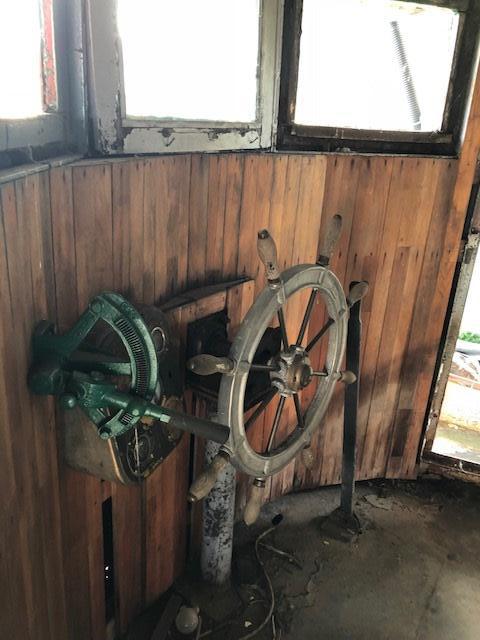This image depicts the inside helm of an old, out-of-commission ship. Dominating the scene is the ship's wheel, a beige-brown apparatus with various spokes, protruding from a central axis that makes steering possible. The wheel is set somewhat low, surprisingly not at eye level, and is supported by a silver pole emerging from wood panels that exhibit age and decay, marked by dark brown spots.

Above the wheel, the structure features three rusted metal-framed windows; the brightness outside contrasts starkly with the worn interior. To the left of the wheel, an intriguing green instrument, akin to a protractor with a handle, is mounted, suggesting it can be moved up and down, possibly as an operational lever for the ship.

The flooring beneath reveals a gray concrete-like surface, littered with dirt and dust, indicating neglect. To the right, a doorway framed in metal leads elsewhere in the ship, reinforcing the appearance of an old vessel that has seen better days and is now partially disassembled.